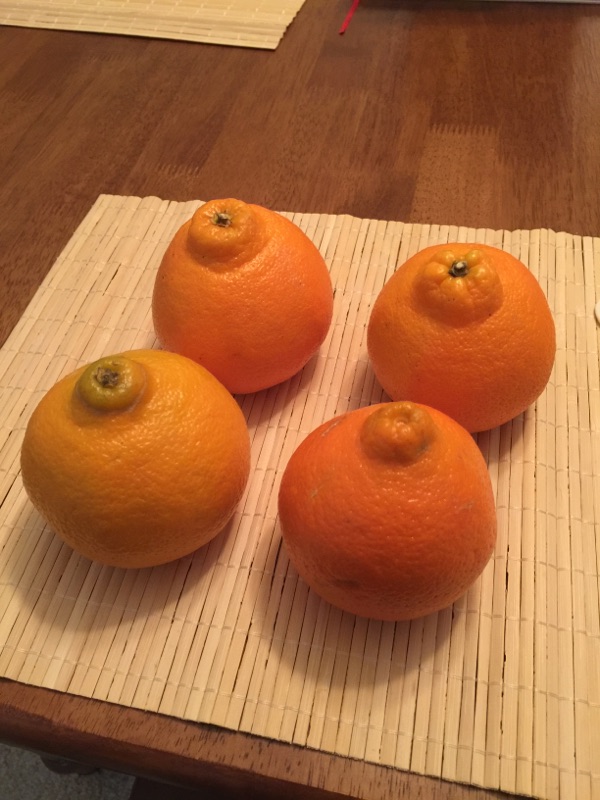This color photograph, taken in portrait orientation, showcases four citrus fruits, likely oranges, placed in the foreground on a light beige bamboo mat with slats, giving it a pliable, foldable appearance. The fruits are arranged two by two on the mat, which in turn is situated on a darker brown wooden table. The table appears slightly angled to the right. The four oranges are nearly identical in size and shape, each with a characteristic navel bump where the stem once was, except for the bottom right orange, which lacks a stem remnant. The bottom left orange is distinguishable by its lighter, yellowish-orange hue, while the remaining three are darker, bright orange. In the upper left corner of the image, you can glimpse another section of a bamboo mat and a mysterious thin red object that extends out of the frame. Additionally, part of the floor, which appears gray, is subtly visible in the bottom left corner of the photo. Shadows cast by the fruits suggest the lighting source is coming from the top right of the image.